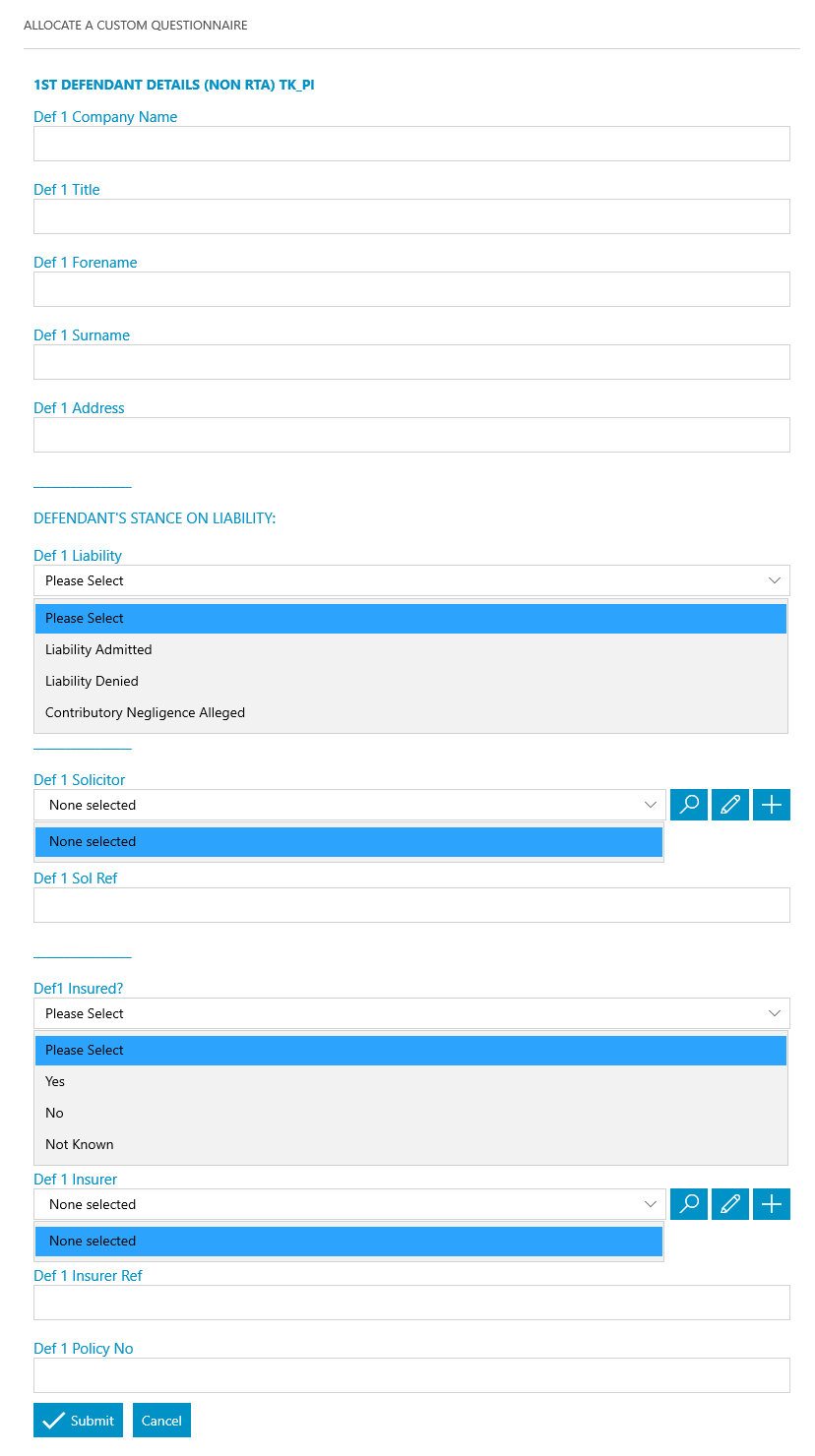This image is a screenshot, likely from a mobile phone or similar device. It depicts a long, narrow webpage interface designed for data entry, featuring a series of fields to fill out. The background is predominantly white with subtle grey outlines defining each field. Labels for these fields are marked in blue. The text throughout the page is exceptionally small, making it difficult to read. The interface is organized into several sections, each separated by blue lines and headers that are just as minuscule as the rest of the text. Some sections have white backgrounds indicating fillable fields, while others have grey backgrounds, indicating non-fillable areas.